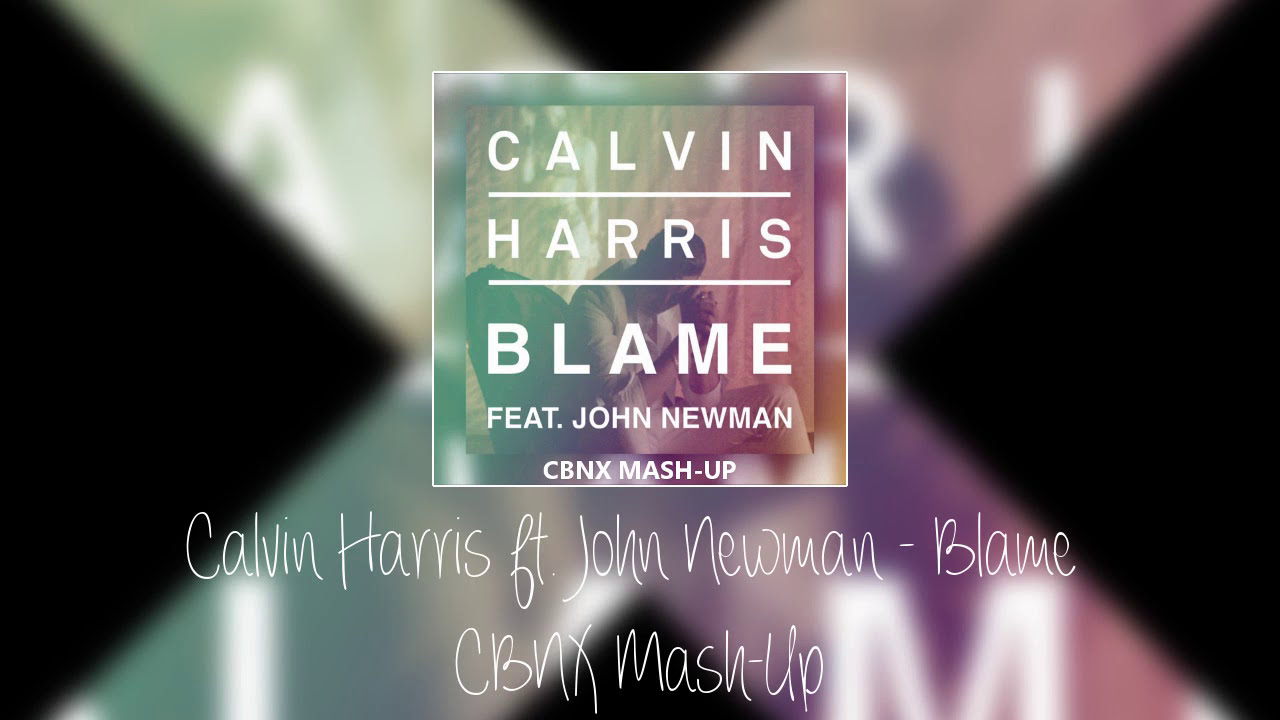This image, which is likely a cover slide for a platform like Spotify or YouTube, showcases the song "Blame" by Calvin Harris featuring John Newman, labeled as a CBNX mashup. The central focus is a large X that spans diagonally across the black background, with vibrant streaks of purple and white. Positioned upward in the center is a square frame, featuring green on the left and top, and purple on the right, with a split of green and purple at the bottom. Inside this square, in white lettering, the text "Calvin Harris, Blame, featuring John Newman, CBNX mashup" is displayed, with the featuring artist and mashup details in smaller font. Behind this text, there's an image of a man, head bowed and hands on his forehead, giving an impression of a contemplative pose. Below this central square, in cursive-like handwritten white script, the same information is repeated: "Calvin Harris featuring John Newman - Blame CBNX mashup." The use of bright colors against the dark backdrop enhances the visibility of the text and the overall aesthetic of the cover.